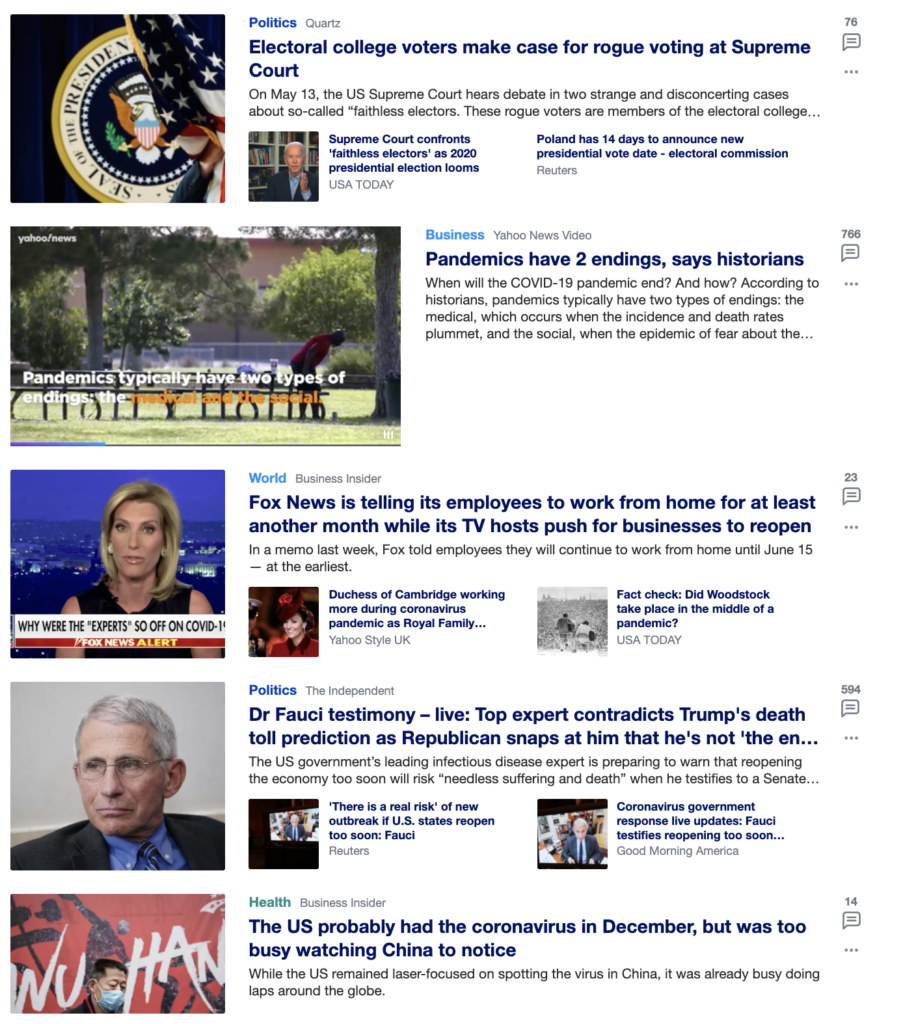The image showcases a collection of news articles and headlines against a predominantly white background with black text and blue clickable links. The top headline falls under the "Politics" and "Courts" sections, reading: "Electoral College voters make case for rogue voting at Supreme Court." The accompanying text notes that on May 13th, the U.S. Supreme Court will deliberate two unusual and troubling cases concerning so-called faithless electors—members of the Electoral College who do not vote in accordance with their pledged candidate. This segment features images of the Presidential Seal of the United States and an American flag.

Below this, under the "Business" section, there's a headline from Yahoo News Video that reads: "Pandemics have two endings, says historians. When will the COVID-19 pandemic end, and how?" It explains that according to historians, pandemics usually conclude in two ways: medically—when new cases and death rates drop significantly—and socially—when the public's fear of the epidemic diminishes. This article is illustrated with a serene image of a park, featuring an open green space with a single person appearing distant and isolated.

At the bottom of the page, another headline states: "The U.S. probably had the coronavirus in December, but was too busy watching China to notice." The text elaborates that while the U.S. was intently focused on detecting the virus in China, it had already begun spreading globally. 

Overall, the layout is clean, featuring news articles in a straightforward format with a focus on current events and insightful analyses.